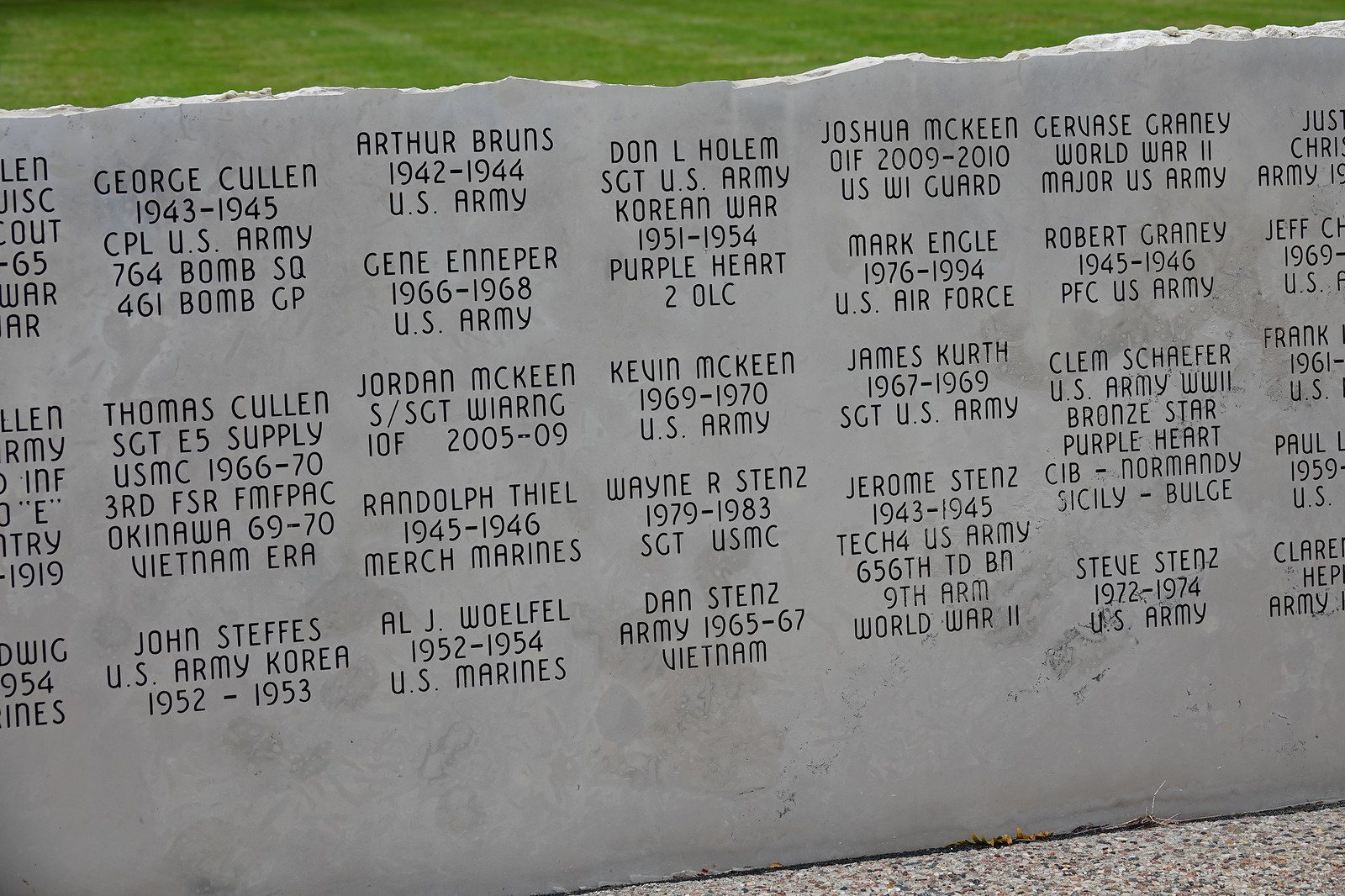The image appears to be of a memorial wall in a military cemetery, displaying the names of numerous fallen soldiers who served in various branches of the armed forces. The wall is a large, jagged piece of gray stone, with black engraved text detailing each individual’s name, the years they served, and their respective military branch. For instance, it features names such as Kevin McKean, who served from 1969-1970 in the U.S. Army, and Arthur Bruns, who served from 1942-1944 in the U.S. Army. The background includes a grassy area, suggesting the memorial is situated in an outdoor setting. The dates of service range widely from the early 1940s to the mid-2000s, covering conflicts like World War II, Vietnam, and the Korean War. The names are listed in no apparent chronological or alphabetical order, and they span various branches including the U.S. Marines, Merch Marines, and even specific roles like Major U.S. Army or Bomb Squad Army. The memorial serves as a solemn tribute to soldiers from different eras and wars.